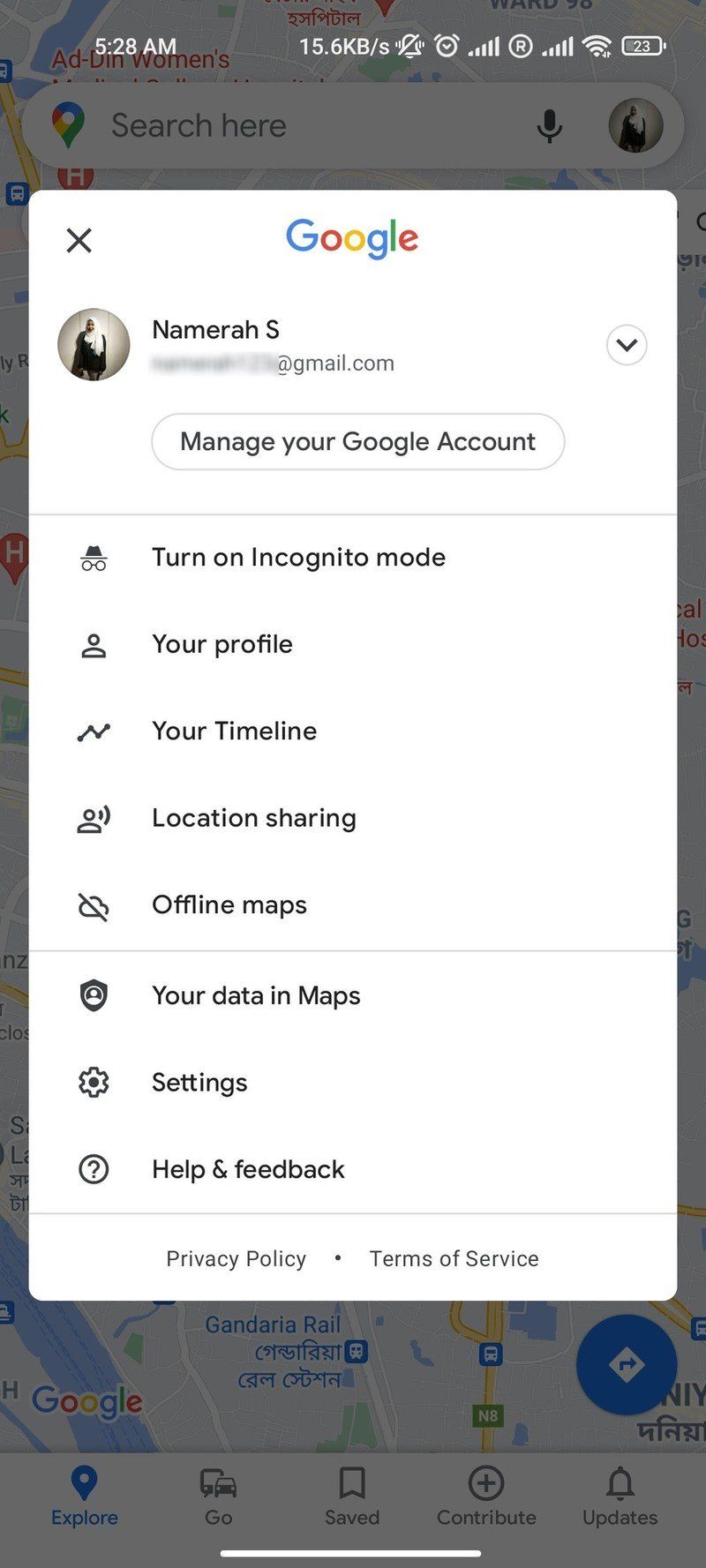The image displays a Google Maps screen on a smartphone, featuring a prominently centered pop-up menu. The top of this menu showcases the colorful Google logo, composed of blue, red, yellow, and green letters. Below the logo, it lists the user’s name, Namera S., with the email address partially blurred, ending in html.com. Following this, an option to "Manage your Google Account" is provided. The menu continues with various options: "Turn on Incognito Mode," "Your Profile," "Your Timeline," "Location Sharing," "Offline Maps," "Your Data in Maps," "Settings," and "Help and Feedback."

The background of the pop-up menu is white, and the text is rendered in black, providing clear readability. At the bottom of the menu, there are links to the "Privacy Policy" on the left and "Terms of Service" on the right.

In the main app interface behind the menu, several navigation buttons are visible at the bottom of the screen, including "Explore," "Go," "Save," "Contribute," and "Updates." "Explore" is highlighted in blue, indicating it is the selected option, while the others are gray. Additionally, a blue circular button featuring a white curved arrow pointing right is located above the "Updates" button. The map visible in the background includes city names such as Kandaria Rail, indicating a railroad location.